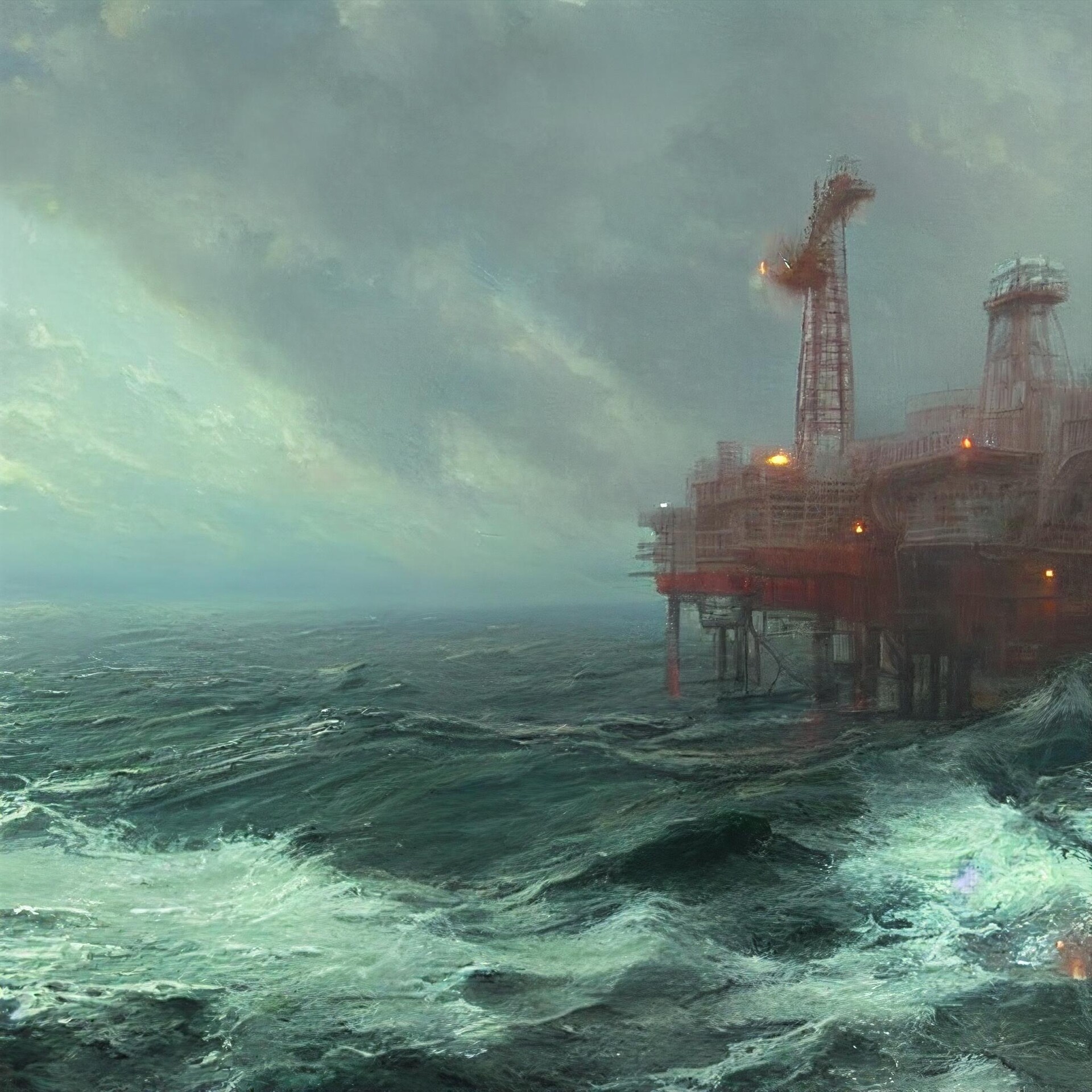The painting depicts a turbulent ocean scene with an oil rig prominently positioned to the right. The hand-painted imagery of the ocean in the foreground showcases rough, volatile waves and white caps, hinting at an impending storm. The sky above is a mix of moody gray clouds with a gradient that fades into blue towards the horizon. The oil rig, adorned with red trim and illuminated by a few reddish lights, includes two prominent towers: a large beacon tower with a light at the top and possibly a water tower. A crane extends from the rig, adding to the industrial feel. The wooden dock, also part of the rig structure, features several lights and a ladder leading up to the taller tower, inviting the eye upwards through the stormy atmosphere. The painting vividly captures the raw power of nature clashing with man-made structures.